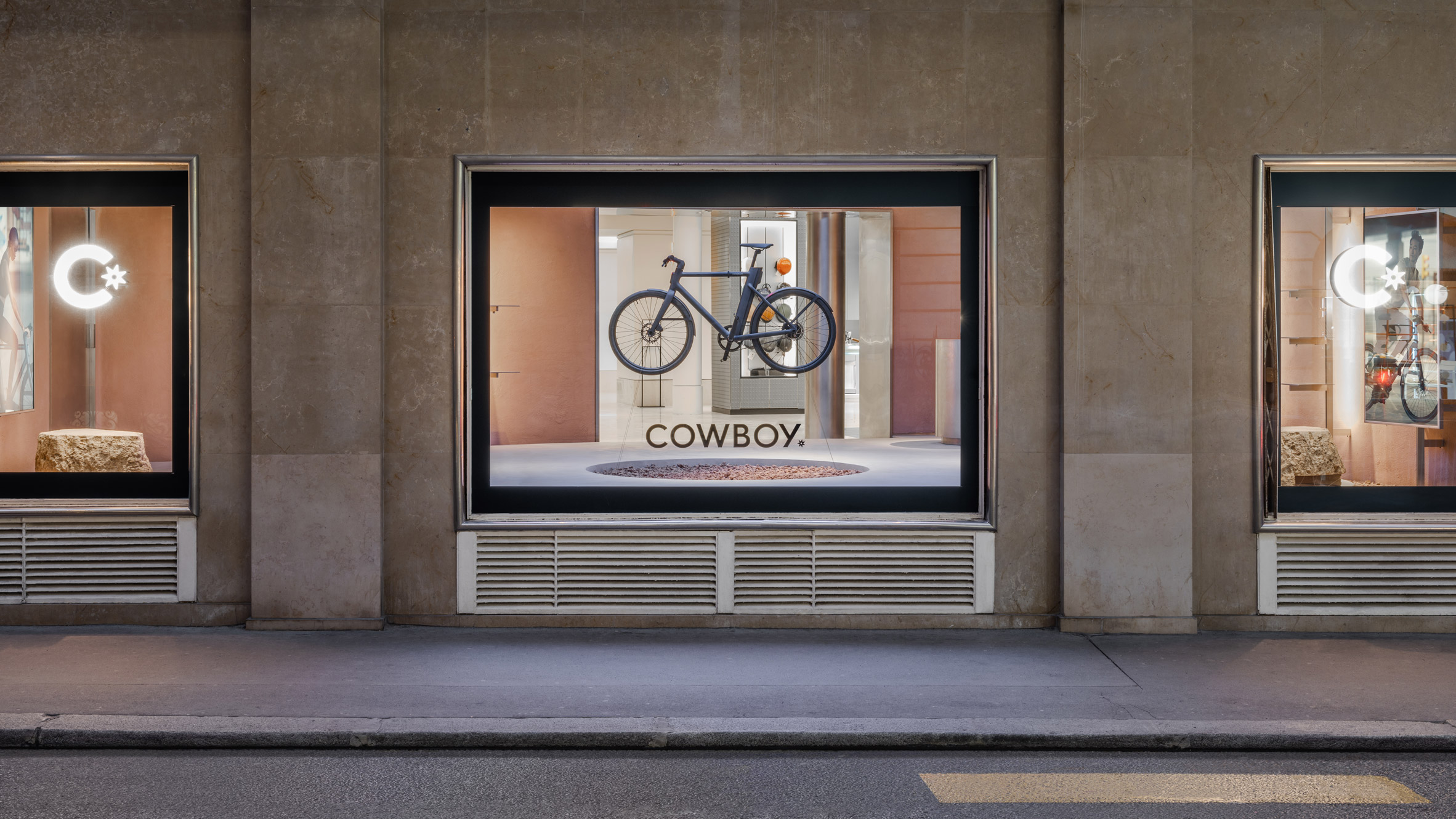This image captures a color photograph of a storefront display window in a brown stone-colored building. The viewpoint appears to be from across the street, incorporating the pavement and a long gray sidewalk in the foreground. The large plate glass window features a bicycle suspended midair against a minimalistic backdrop. The display is framed by a silver border and black frame. At the bottom of the window, the word "Cowboy" is prominently displayed in large brown letters. Inside the window, a circular concrete pit filled with gravel can be seen, along with orange-colored walls that are made of wood.

Flanking the main display window are two partially visible windows, each adorned with a neon white "C" accompanied by a star, presumably the logo for Cowboy. The left and right side windows house similar logos and are part of the same minimalist, modern aesthetic. The vibrant yet neutral color scheme extends throughout the store display, contributing to its contemporary and clean design. Additionally, the interior walls seen through the display are dark brown, enhanced by posters depicting people riding bicycles, further emphasizing the store's focus on cycling.